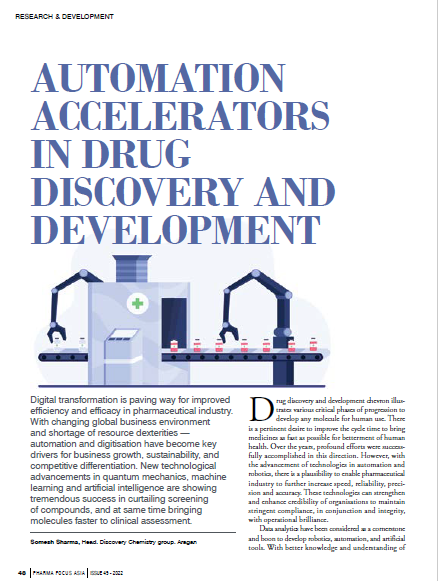The image appears to be a page from a magazine article focused on advancements in the pharmaceutical industry. At the top left, in small black letters, it reads "Research and Development," followed by a prominent title in bold, all-caps, blue font: "AUTOMATION ACCELERATORS IN DRUG DISCOVERY AND DEVELOPMENT." Below this title, the main visual is an infographic depicting a factory assembly line. The machine in the image has two claw-like structures on either side. On the left, it moves empty bottles onto a conveyor belt, which then passes through a rectangular chamber marked with a green cross. Bottles come out filled with a red liquid on the right, where another claw structure manages them. Additional writing beneath the image provides further description of the depicted process. The overall design features a blue theme and cartoonish art style. A summary blurb on the left talks about digital transformation and its impact on efficiency and efficacy in the pharmaceutical industry, addressing aspects such as business growth and sustainability. Article text continues on the right, and the bottom left corner is marked with the page number 48.